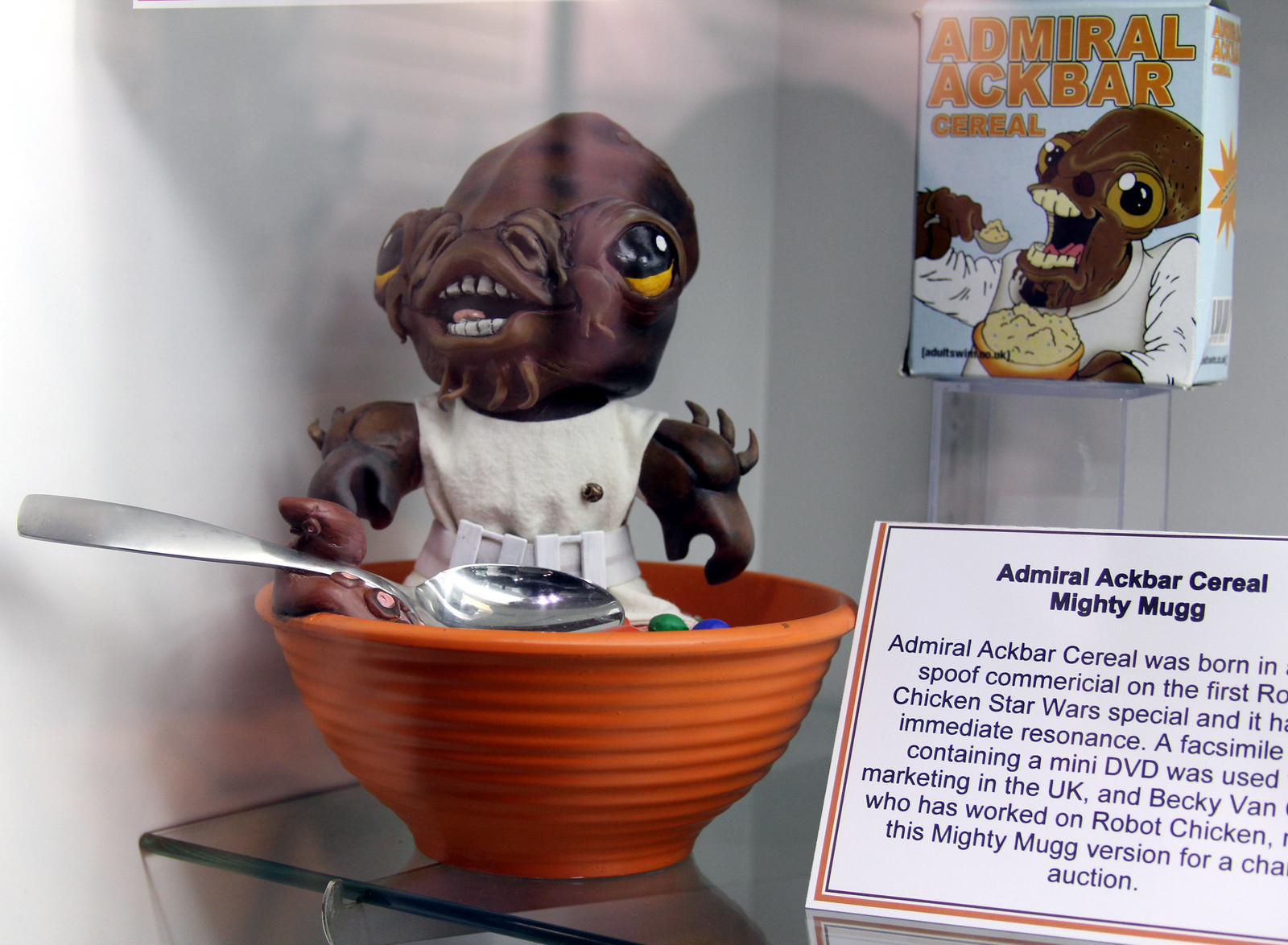This is a wide rectangular image displaying a humorous scene in a glass display case. The background is a light gray wall with glass shelves. The central focus is an Admiral Ackbar toy, a character from Star Wars, with a brown, elongated, octopus-like head, large yellow and black eyes, and a mouth open to reveal white teeth. The figure, dressed in a white sleeveless shirt and belt, resembles a Funko Pop-sized toy and is holding an orange bowl of cereal with a silver spoon in front of it. 

Behind the toy, on the upper right corner, there's a box labeled "Admiral Ackbar Cereal" showing a cartoon illustration of Admiral Ackbar eating cereal with a spoon. The box features a smaller inscription for adultswim.com.uk. Below the toy, there is a plaque that partially reads "Admiral Ackbar Cereal, Mighty Mug" with the following incomplete text: "Admiral Ackbar Cereal was born in... spoof cereal commercial on the first Chicken Star Wars special... immediate resonance... containing a mini DVD... used in marketing in the UK... Becky Vann who has worked on Robot Chicken... Mighty Mug version for auction." The entire scene seems to be a playful display related to a spoof commercial from the Robot Chicken show.